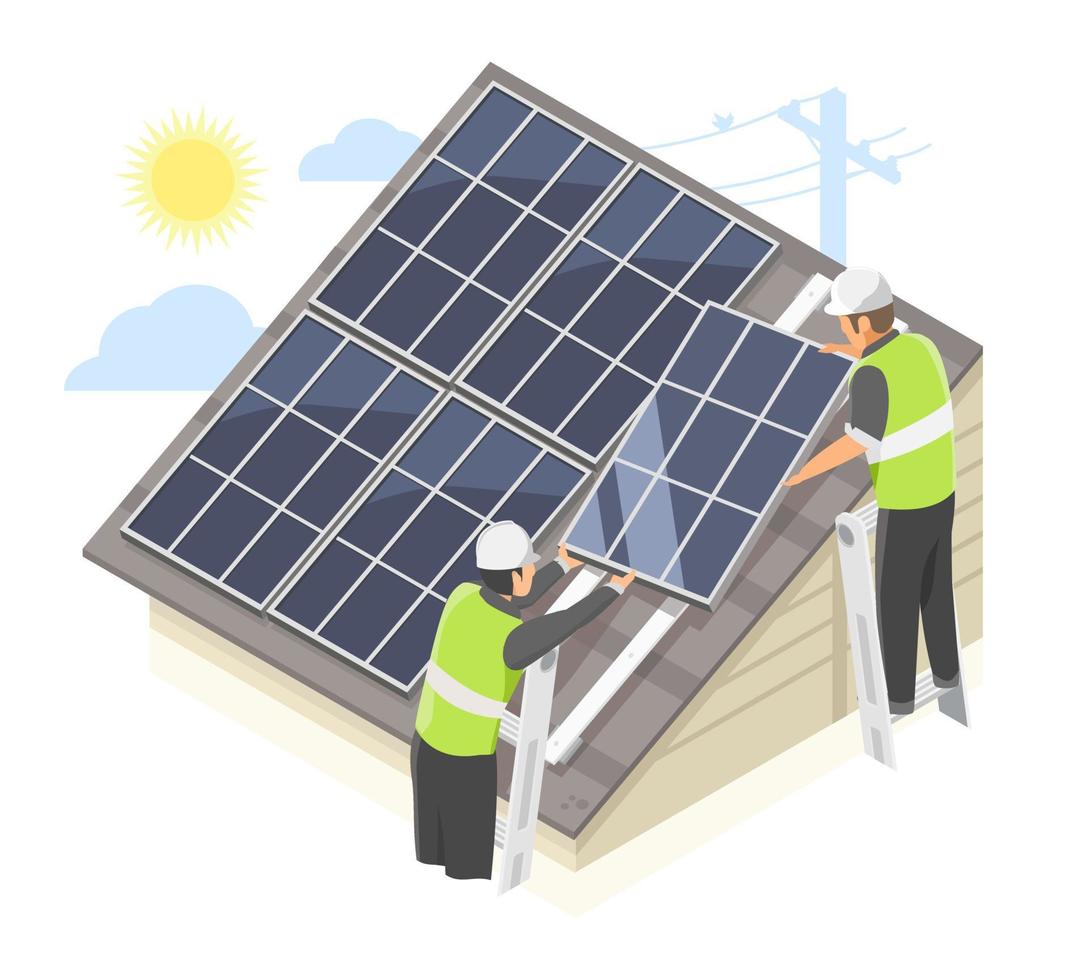In this cartoonish illustration, two men are installing solar panels on a slanted, light brown roof. Both workers are dressed in white helmets, gray suits, and light green safety vests with white stripes. They stand on separate white extension ladders, collaboratively handling a nine-paneled solar section that is grey with white dividing lines, adding it as the fifth of six sections to complete the array. The roof shows four already-installed sections, each arranged into three columns and two rows. In the upper-left corner, a stylized sun with numerous triangular rays radiates, while two light blue clouds float nearby. The upper-right features a light blue telephone pole with wires spanning both sides and a small, light blue bird perched on one wire. The simple white background offers a clean, unobtrusive backdrop to the detailed scene.